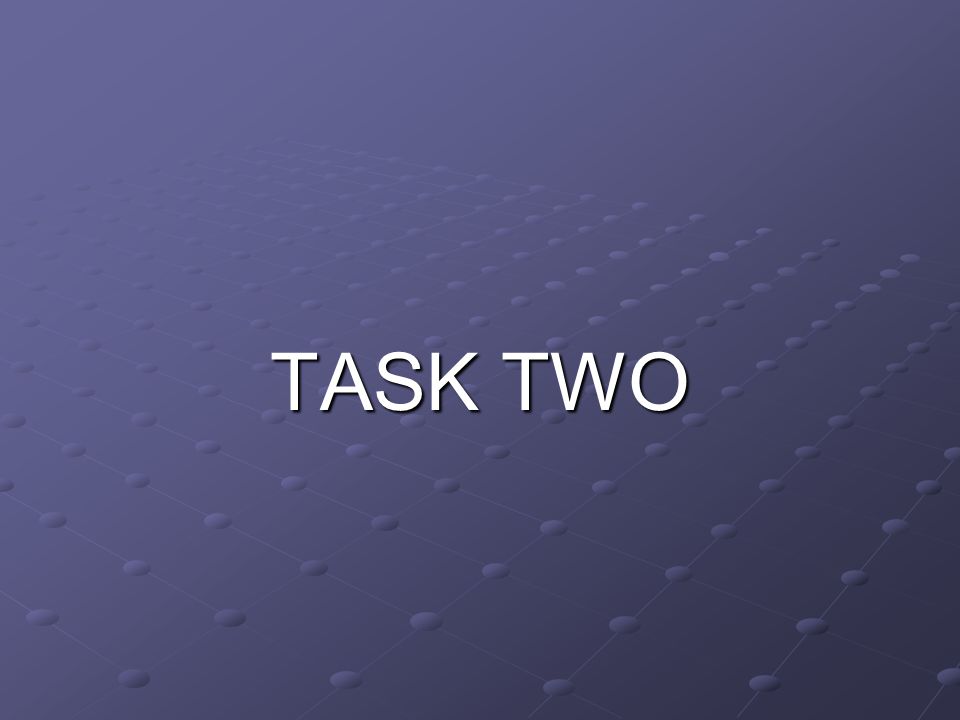The image is a slide from a PowerPoint presentation featuring a visually striking background composed of a purple gradient that transitions from a lighter hue in the top left to a deeper shade in the bottom right. In the foreground, large text reading "TASK 2" is prominently displayed in an all-caps, Times New Roman font, rendered in white with a subtle black drop shadow for added depth. This text is centrally positioned. Behind the text, an intricate graphical pattern of small, raised dots connected by diagonal lines spans the background. These lines run northeast and southeast, forming a grid-like structure. The dots have a slightly shadowed effect, enhancing their three-dimensional appearance against the gradient backdrop. The overall design features a blend of modern aesthetics with a classic font, creating a visually engaging slide that effectively draws attention to the main task.